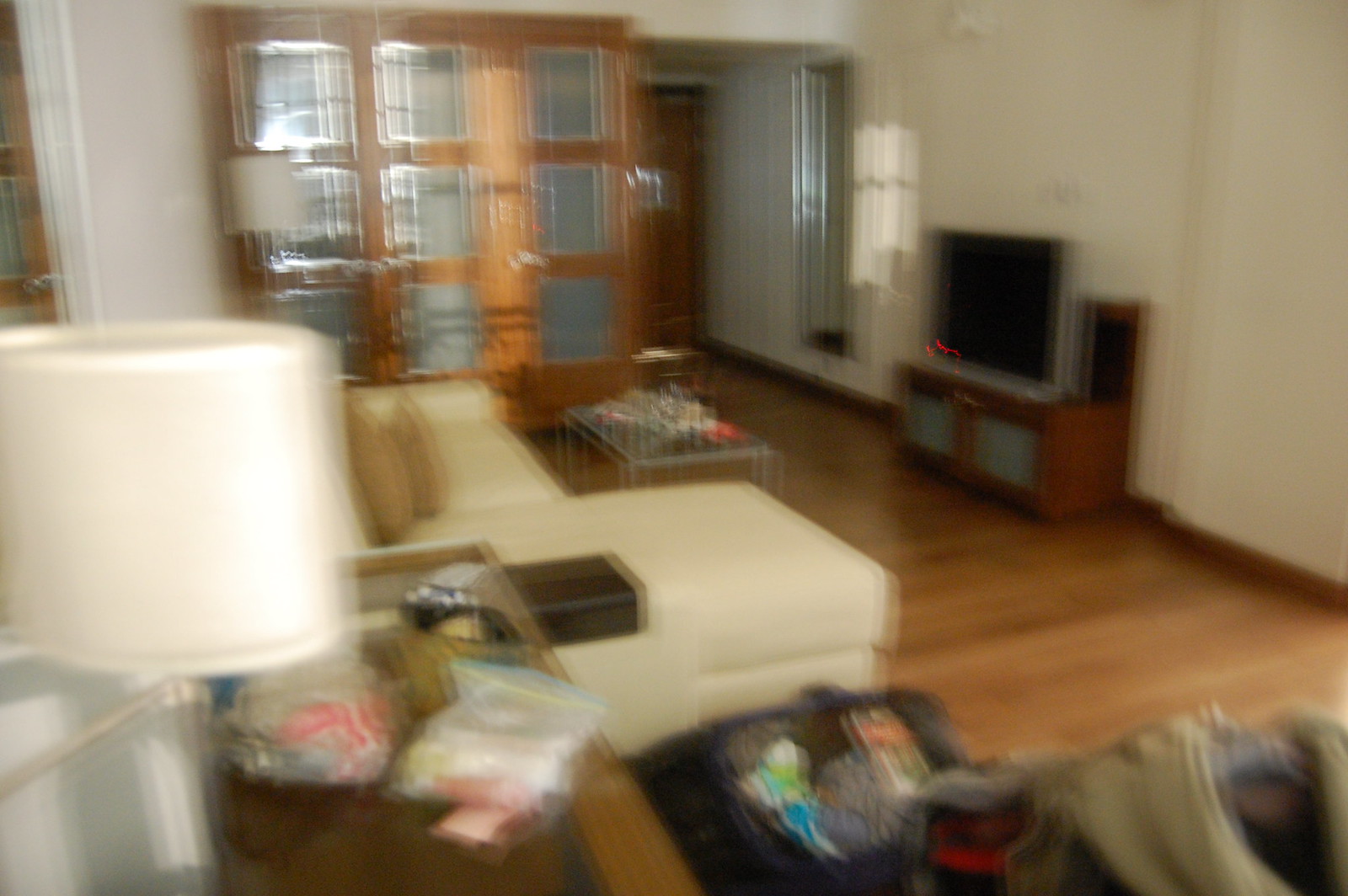This photograph captures a blurry interior of a home, possibly a family room. In the foreground, a light brown wooden tabletop, likely a dresser or table, hosts a cream-colored lampshade surrounded by clutter, including a crumpled plastic bag with red writing, a Ziploc bag, and various receipts and papers. A blocky, cream-colored sofa with light tan throw pillows sits prominently in the mid-ground, accompanied by a silver or light gray framed coffee table piled with debris. Further back, a dark brown hutch featuring two doors with light gray centers supports a large black flat-screen TV, which displays a red digital clock in the bottom left corner. The far end of the room reveals a white-brown colored door adorned with silver-framed, square-shaped glass panels. Adjacent to this door is an indentation for a tall, rectangular window. The walls are white, and the flooring is light tan wood, adding to the home's somewhat disorganized yet cozy ambiance.